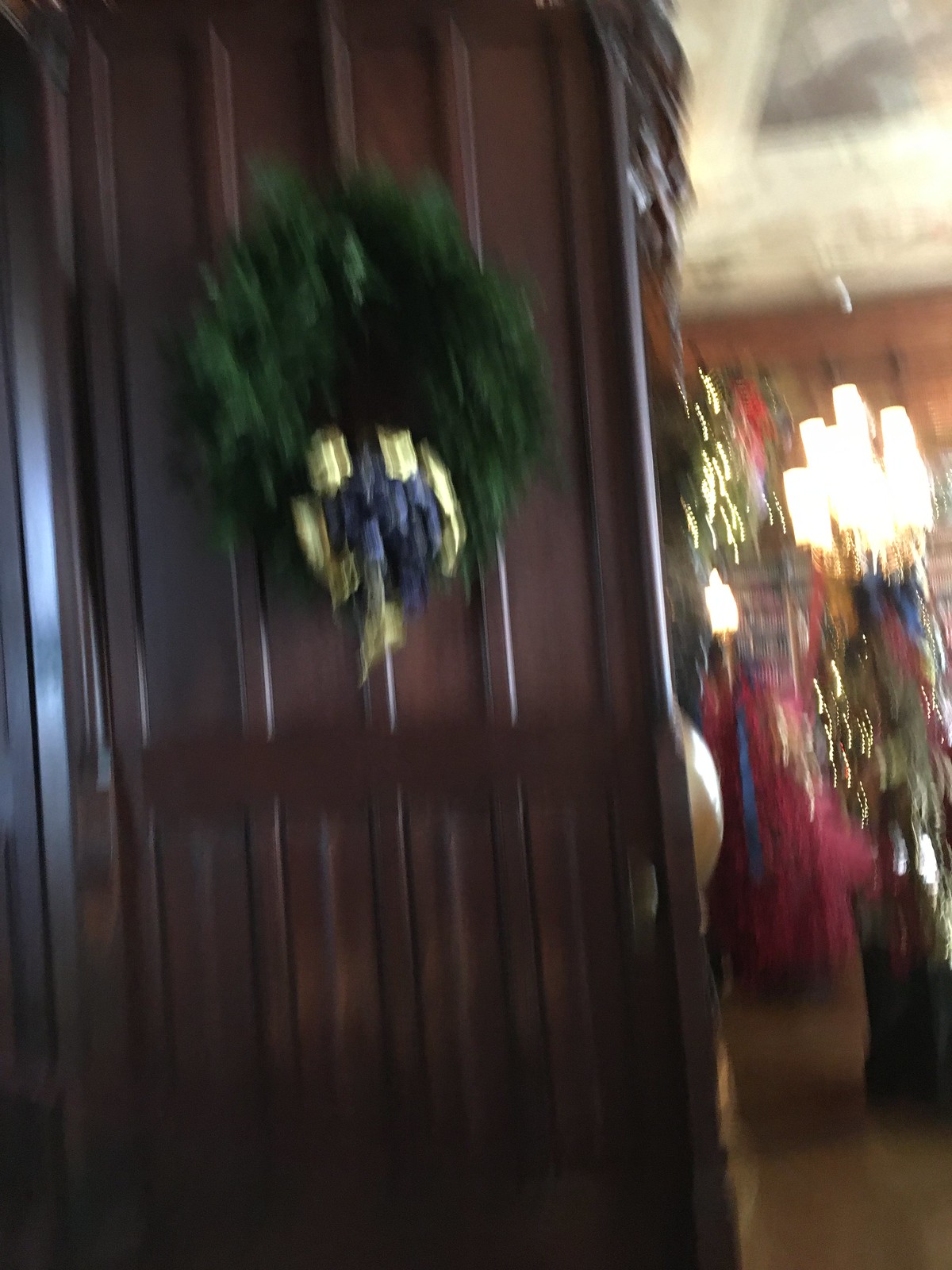This blurry image captures what appears to be a festive indoor scene, possibly taken inadvertently. Dominating the left side is a large dark brown front door with decorative lines, made of wood that borders on a cherry color. The door is adorned with a green Christmas wreath, which features a gold and blue bow tied at its bottom. To the right of the wreath, a bright pendant light stands out, though it appears blurry due to the quality of the photograph. Additionally, to the left of the light, another green wreath decorated with bright white Christmas lights can be seen. Below the light, there is a visible red chair, and in the background, there seems to be a bookcase filled with books. The image also includes a mix of colors and lights, contributing to a festive atmosphere that suggests it was taken during Christmastime.